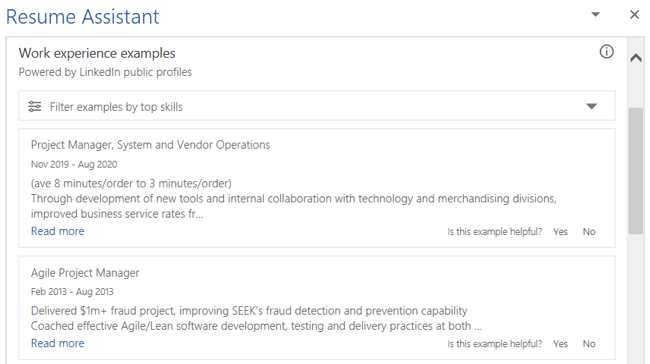This monochromatic screenshot, likely from a website or application, features a white background with dark gray text. At the top, the header reads "Resume Assistant" in blue text. To the right of this header, there is a dropdown menu arrow and an "X" to close the window. Below the header, a box with gray lines demarcates the top and left sides. Inside this box, the title reads "Work Experience Examples," accompanied by a note stating "Powered by LinkedIn public professionals." Directly beneath this, a filter box allows users to narrow examples by top skills, with a dropdown arrow on the right side of the box.

Further down, the screenshot displays part of a person's resume. The first entry lists "Project Manager, System and Vendor Operations" with the date range "November 2019 to August 2020." The second entry is titled "Agile Project Manager" with the date "February 2013 through August 2013."